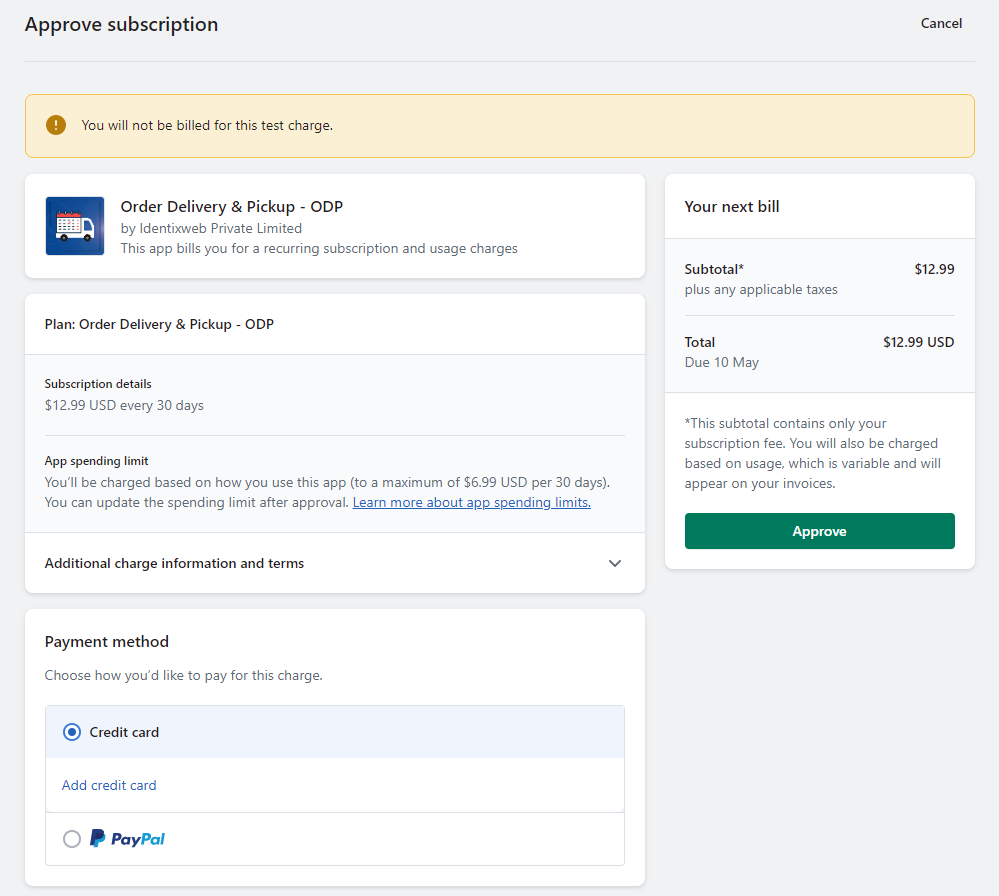The image is a webpage designed for the approval of a subscription, featuring a tan-colored background. At the top of the page, the title "Approve Subscription" is displayed on the left, accompanied by a "Cancel" button on the right. Just below this, there is an orange-brown alert box with an exclamation mark and the message, "Attention: You will not be billed for this test charge."

Below the alert box, a white rectangular section with a delivery truck icon reads, "Order Delivery and Pickup - ODP by Identix Web Private Limited. This app bills you for recurring subscription and usage charges." 

Further down, there are four additional white boxes containing black text:
1. **Plan**: "Order Delivery and Pickup - ODP."
2. **Subscription Details**: "$12.99 U.S. every 30 days."
3. **App Spending Limit**: "You'll be charged based on how you use this app, up to a maximum of $6.99 USD per 30 days. You can update this spending limit after approval" with a link to "Learn more about App Spending Limits."
4. **Additional Charges and Information**: A drop-down arrow indicating further details.

The final white box outlines the **Payment Method**. Users can choose how they'd like to be billed for the charge, with two options:
- A radio button for **Credit Card** (currently selected) along with an "Add a Credit Card" link.
- A radio button for **PayPal** (not selected).

On the right side of this section, a summary box titled **Your Next Bill** shows the following:
- **Subtotal**: $12.99
- **Total Due Date**: 10 May, amounting to $12.99 USD.
A note clarifies: "This subtotal contains only your subscription fee. You will also be charged based on usage, which is variable, and will appear on your invoices."

Finally, at the bottom of the section, there is a prominent green "Approve" button.